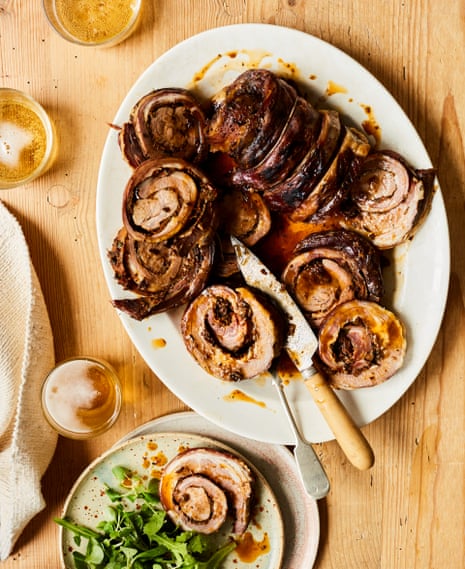In this overhead photograph, we see a well-prepared pork roast dinner displayed on a light blonde wooden table. The focal point is a white ceramic oval platter that holds a sliced pork loin rolled and tied with string before cooking, featuring a dark brown exterior and lighter pink interior. The meat, cut into pinwheels, is draped in a rich brown gravy. Adjacent to this, in the bottom left, sits a speckled green and brown pottery plate containing a spiral cut of the pork alongside a fresh arugula salad. Three clear glasses of amber liquid, possibly beer, are also present; one near the bottom left of the image and two in the upper left corner. Partially captured on the left side is a white canvas mat, adding a hint of texture to the scene. A serving knife rests on the white platter, ready for further carving.